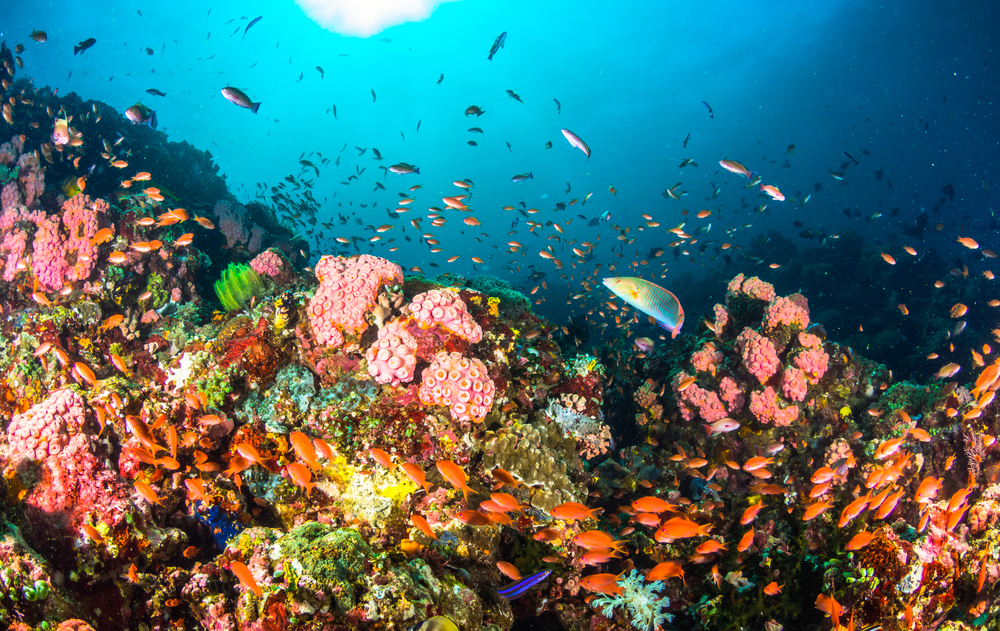The vibrant underwater scene captures a thriving and dynamic coral reef teeming with life. The coral reef is a dazzling array of colors, featuring shades of pink, red, green, blue, and yellow. Various species of colorful coral protrude from the reef, with bright pink and red corals standing out prominently. A large school of orange fish swims over and around the coral, mingling with other fish of different hues, including some striking blue ones. In the clear, deep blue water that stretches into the background, there are countless bait-sized fish schooling together, contributing to the sense of a bustling underwater habitat. The water is well-lit, revealing detailed textures and the multitude of marine life thriving in this vibrant ecosystem. Adding to the diversity, a peculiar, strange-looking blue fish, possibly an eel, is seen emerging from a crack in the coral. Overall, this bright, colorful image portrays a very active and flourishing coral reef, with hundreds of fish in various shapes and sizes moving in harmony within this underwater paradise.